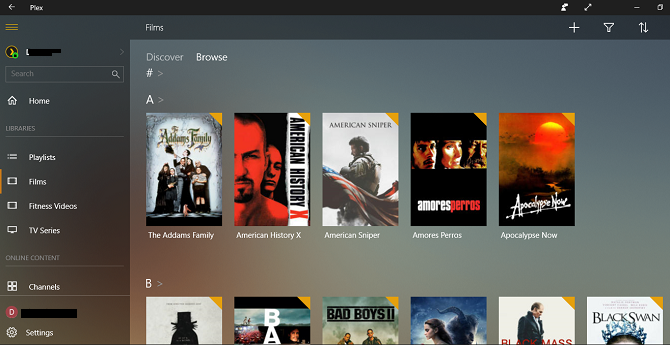The image depicts a window of an unidentified application or program, which closely resembles the interface of iTunes but lacks a clear title. In the upper left corner, there is a back arrow for navigation, followed by a blurred text that possibly reads "Pink" or "Pics." The upper right corner features several icons: a maximize button, an icon of a person with a chat bubble that might represent a chat function, a minimize button, and an additional indistinguishable button.

On the left-hand side of the screen, below the back arrow, there are three horizontal bars indicating a menu option. Below this, there is a profile picture with an associated name that is obscured. Directly beneath the profile, there is a search bar. Continuing down the left side, the menu options listed include: Home, Playlists, Films, Fitness Videos, and TV Series buttons. Further down, the menu displays options for Online, Continue (possibly truncated), Channels, another obscured name, and Settings.